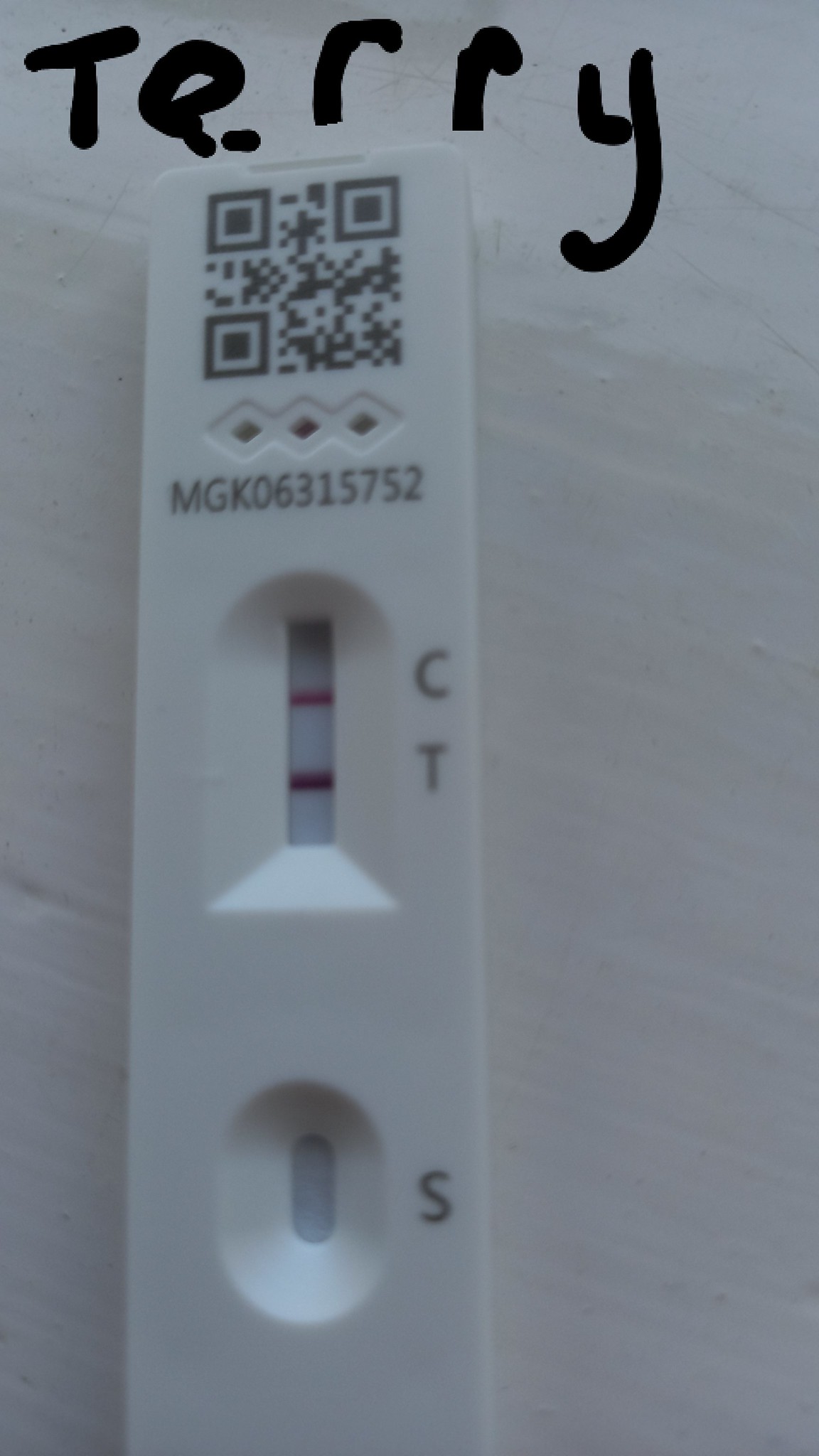This photograph features a unique, digitally altered image. The base image appears to be a photograph of some sort of rectangular device placed on a white surface. Overlaying this photograph are various elements seemingly drawn in Microsoft Paint.

In the photo's lower section, there is a prominent black, uppercase "S" to the right of a circular plug with a single gray tab in its center. Above this plug, the letter "C" sits, and directly below, the letter "T," both in uppercase, arranged vertically.

To the left of this setup, there is another set of overlays resembling the earlier circular plug but featuring three gray tabs instead of one. This object has a distinctive shape, reminiscent of a rocket, with a smooth, rounded top and a square bottom.

At the very top of the photograph, a QR code is visible, with a typical square arrangement and notable dark squares in the top-left, top-right, and bottom-left corners, surrounded by a pattern of black dots and white spaces.

Additionally, the entire image is framed with black ink drawings using MS Paint, prominently featuring the name "Terry" at the very top, suggesting the creator or annotator of the image.